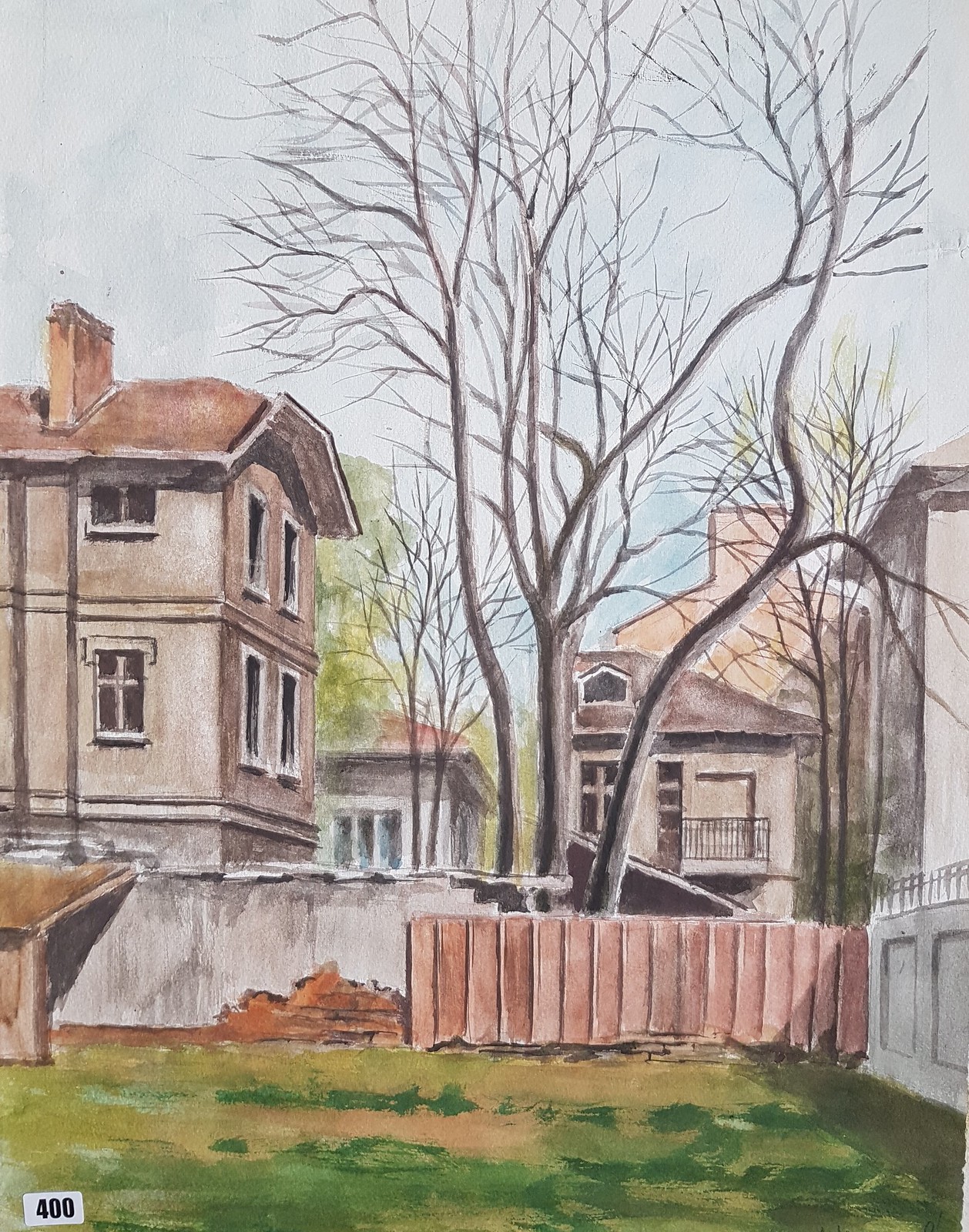A detailed illustration of a suburban backyard is depicted within a fenced-in area. The right side features a classic white fence, while the front has an orange-brown barrier transitioning into a gray concrete wall approaching the adjacent property. A pile of brown material, possibly firewood, is stacked nearby. The ground displays a flat, greenish-brown lawn, devoid of individual grass strands but painted with a uniform color. In the bottom left corner, a white sticker with the number "400" in black text is visible. Bare, brown trees with branching limbs populate the middle ground, adding a touch of natural complexity. Prominent on the left side, and scattered in the background, are several tan houses, each marked by white-bordered windows and reddish-brown roofs, creating a harmonious neighborhood setting.